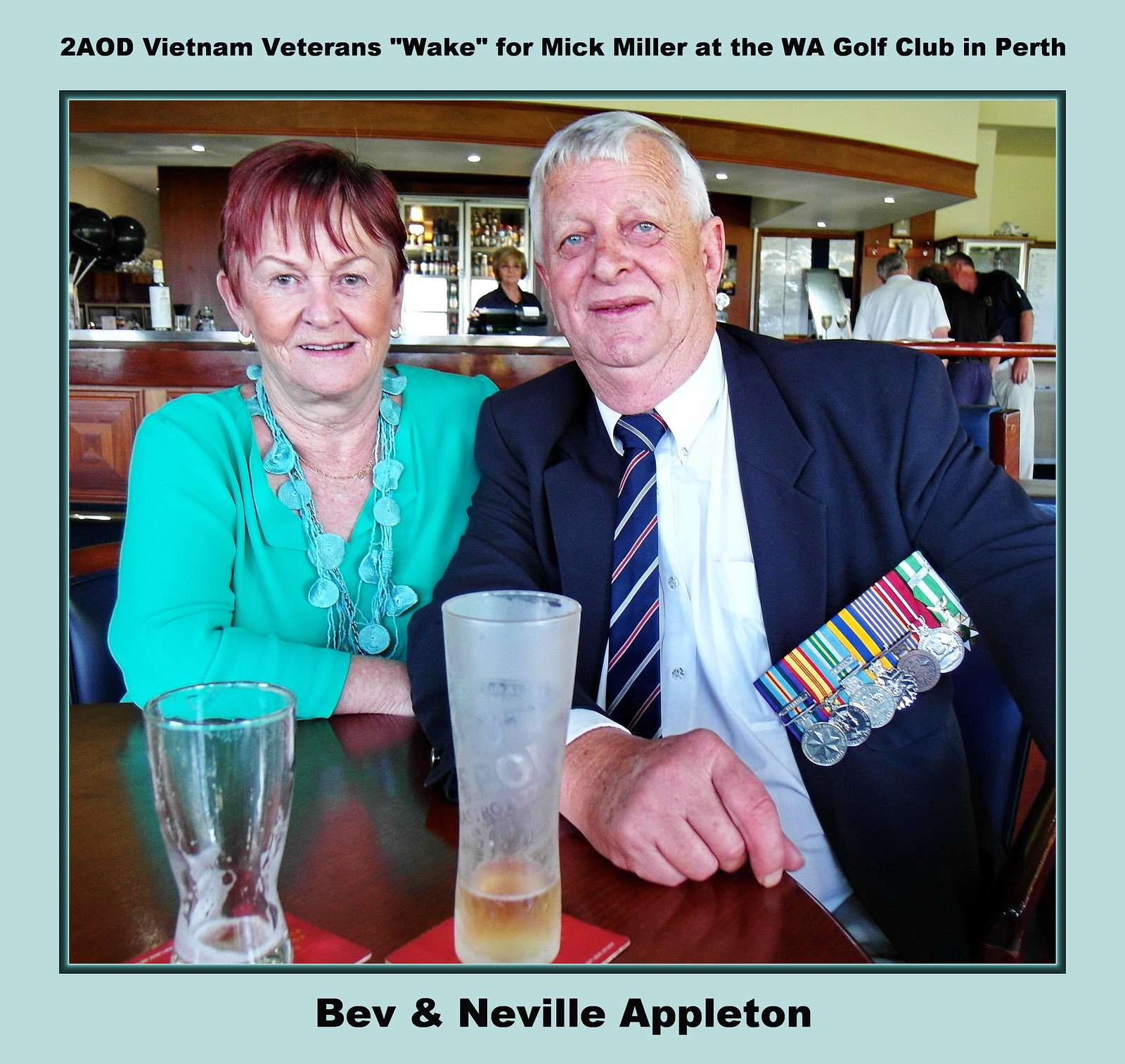The image is a color photograph set within a horizontally aligned, rectangular frame of pale aqua with a blue border. The photo captures two elderly individuals sitting at a table in a bar. In the photograph, a woman in her 60s with short, fringy red hair, wearing a turquoise long-sleeve blouse and matching necklace, smiles warmly at the camera. Seated next to her on the right is a man in his 60s with short gray hair, blue eyes, and a stout build. He is dressed in a white shirt, a white, red, and blue striped tie, and a navy blue blazer adorned with a row of silver military medals and their respective ribbons. Both have their hands resting on the table, which features two beer glasses on red square coasters—one mostly empty and one completely empty. In the background, a mahogany bar with an indoor roof and built-in lights can be seen, along with a Caucasian female bartender and several patrons. Above the photograph, black text reads, "Two AOD Vietnam Veterans 'Wake' for Mick Miller at the WA Golf Club in Perth," and below, "Bev and Neville Appleton" is inscribed in matching black text.